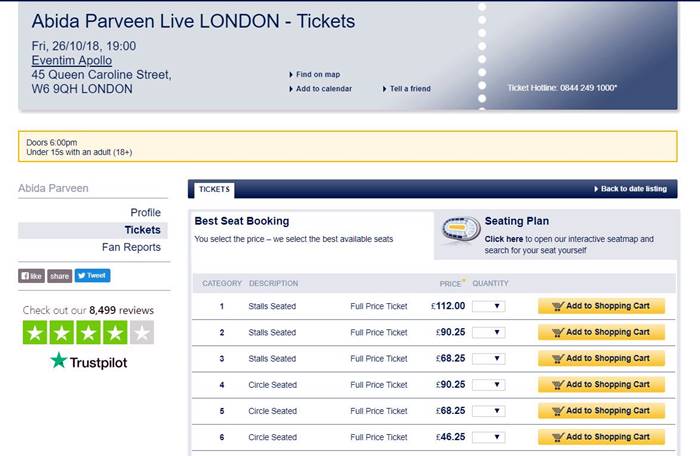This is an image of a ticket booking page for an event titled "Happy Da Praveen Live." The event is scheduled to take place in London on Friday, October 26, 2018, at 7:00 PM at the Eventum Apollo, located at 45 Queen Caroline Street, W6 9QH, London. There is a "Find on Map" button for directions, an "Add to Calendar" option for convenience, and a "Tell a Friend" feature for sharing the event. The ticket hotline number is provided as 0844-249-1000 for additional inquiries. 

A yellow label indicates that doors will open at 6:00 PM and notes that attendees under the age of 15 must be accompanied by an adult aged 18 or older. The banner also mentions "Abada Praveen." 

Additional features on the page include options to view the artist's profile, look at available tickets, or read fan reports. It proudly displays a Trustpilot rating of 4 out of 5 stars, based on 8,499 reviews. 

The ticket booking system offers a "Best Seat Booking" feature, where users can select a price and the system will choose the best available seats. There are six different seating categories, split between stall seats and circle seats. Ticket prices vary, with the most expensive seats priced at £112, and other options available for £90.25, £68.25, and the lowest at £46.25.

The page predominantly features a white background with blue text and assorted images, providing a clean and organized layout for easy navigation and booking.